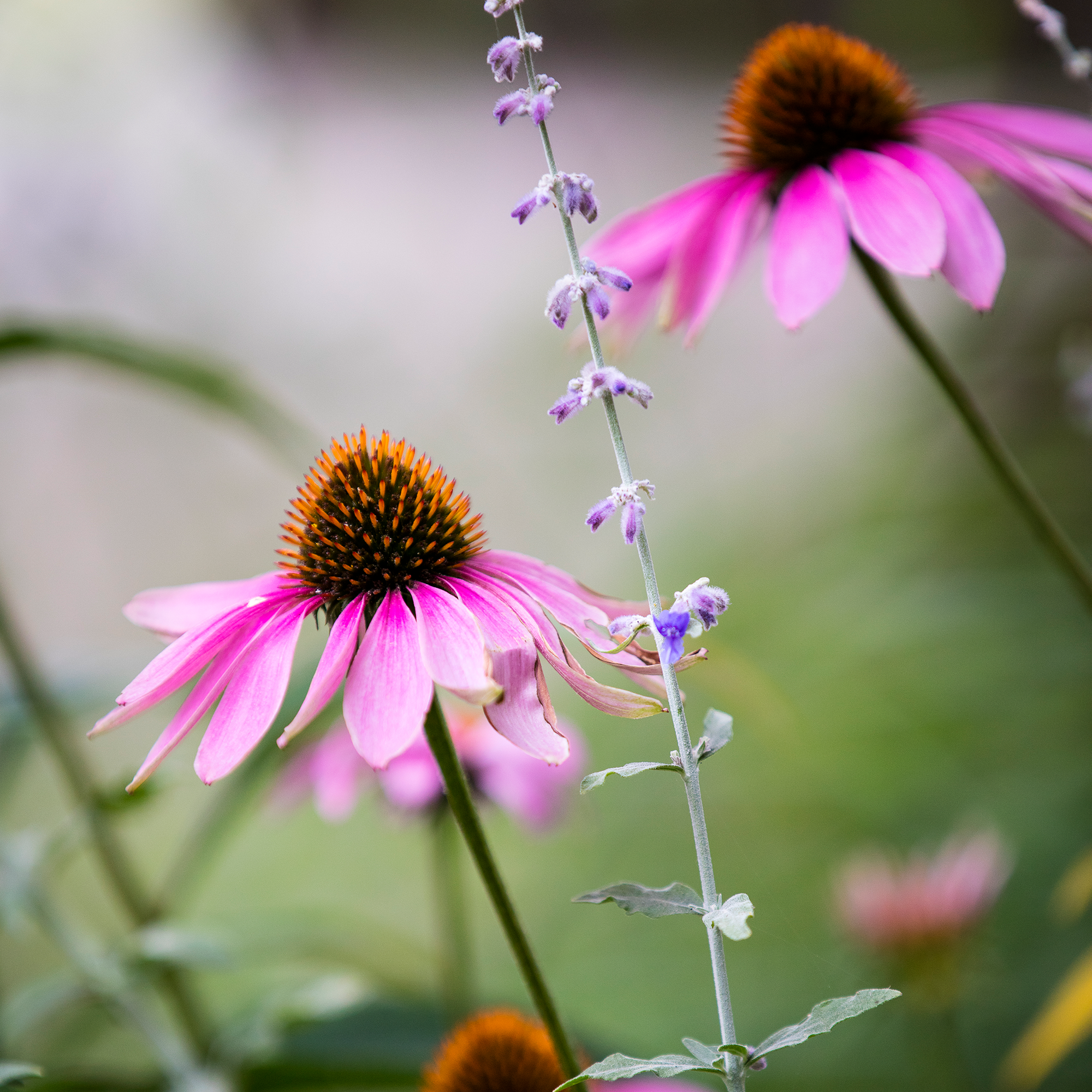This is a close-up image capturing a vibrant garden scene with an emphasis on three vividly detailed Echinacea flowers prominently displayed in the foreground. The flowers feature drooping, pink-purple petals and an orange, spiky stamen resembling a chocolate cream drop in shape and texture. The central Echinacea has a long stem punctuated with tiny pink flowers or buds. Surrounding these primary blooms, the background is artistically blurred, infusing the image with soft hues of green and white light, suggestive of other plants and foliage during daytime. The blur enhances the intricate details of the flowers in focus, making the scene appear serene and inviting, like a haven for pollinators. Additionally, a sprig of lavender, not fully in bloom, interjects vertically in the composition, its delicate purple flowers adding a contrasting charm to the overall floral display. The image radiates a natural beauty and tranquility, capturing a quintessential moment in a lush, sunlit garden.